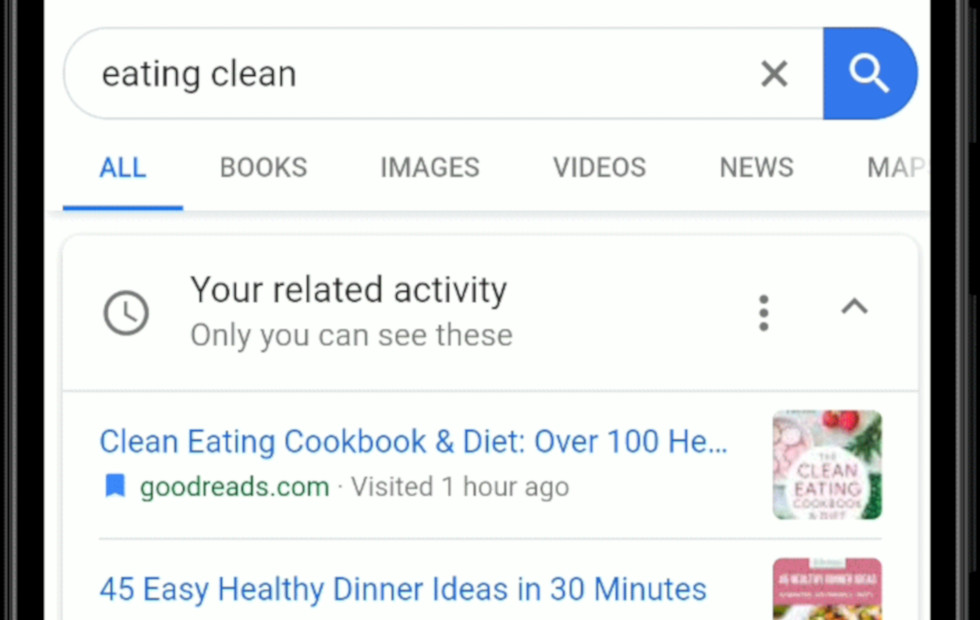Screenshot of a Google search results page for the query "eating clean." The search box at the top shows "all" selected among the options: books, images, videos, news, maps. Below the search box is a section labeled "Your related activity," followed by the note "Only you can see these" with three green dots on the right side. The first search result is from Goodreads.com, visited an hour ago, featuring "Clean Eating Cookbook and Diet." The listing includes a partial view of the book cover and the text snippet "over 100 HE..." before it cuts off. The next result highlights "45 easy, healthy dinner ideas in 30 minutes," though the full description is not visible. This screenshot suggests using a dedicated recipe book for planning clean meals, streamlining the process of gathering ideas and creating grocery lists, and implies that the user has explored multiple resources to gain new insights into clean eating.